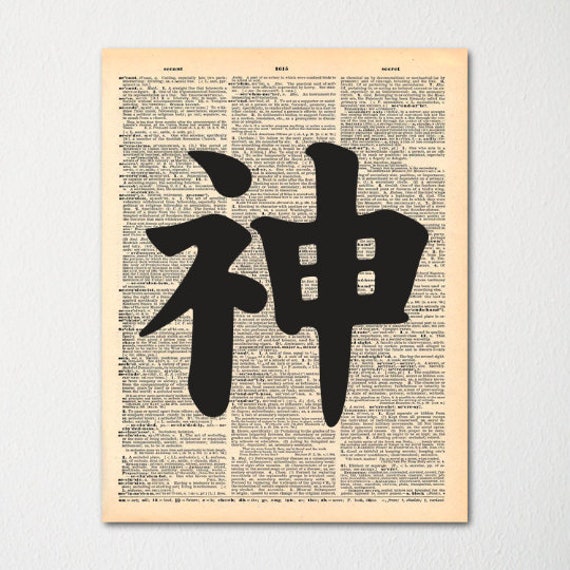The image portrays an aged document resembling an old dictionary page, set against a gray background. The paper is yellowed with time, particularly more so around the top, bottom, and right side, though the left side remains somewhat less discolored. The document is divided into three columns, each containing about 15 bolded words with definitions listed beneath them. Central to the document are large, black Asian script symbols, possibly Chinese or Japanese. The symbols are bold and prominent, with one resembling a line with a water drop at the top and a checkmark, another with a straight line through it, a box in the middle, and two open squares on each side. The third symbol appears like a Z with a line at the bottom. The background text is in a small font and blurry but structured like paragraphs, lending the entire piece the appearance of a historical text overlayed with striking calligraphy.